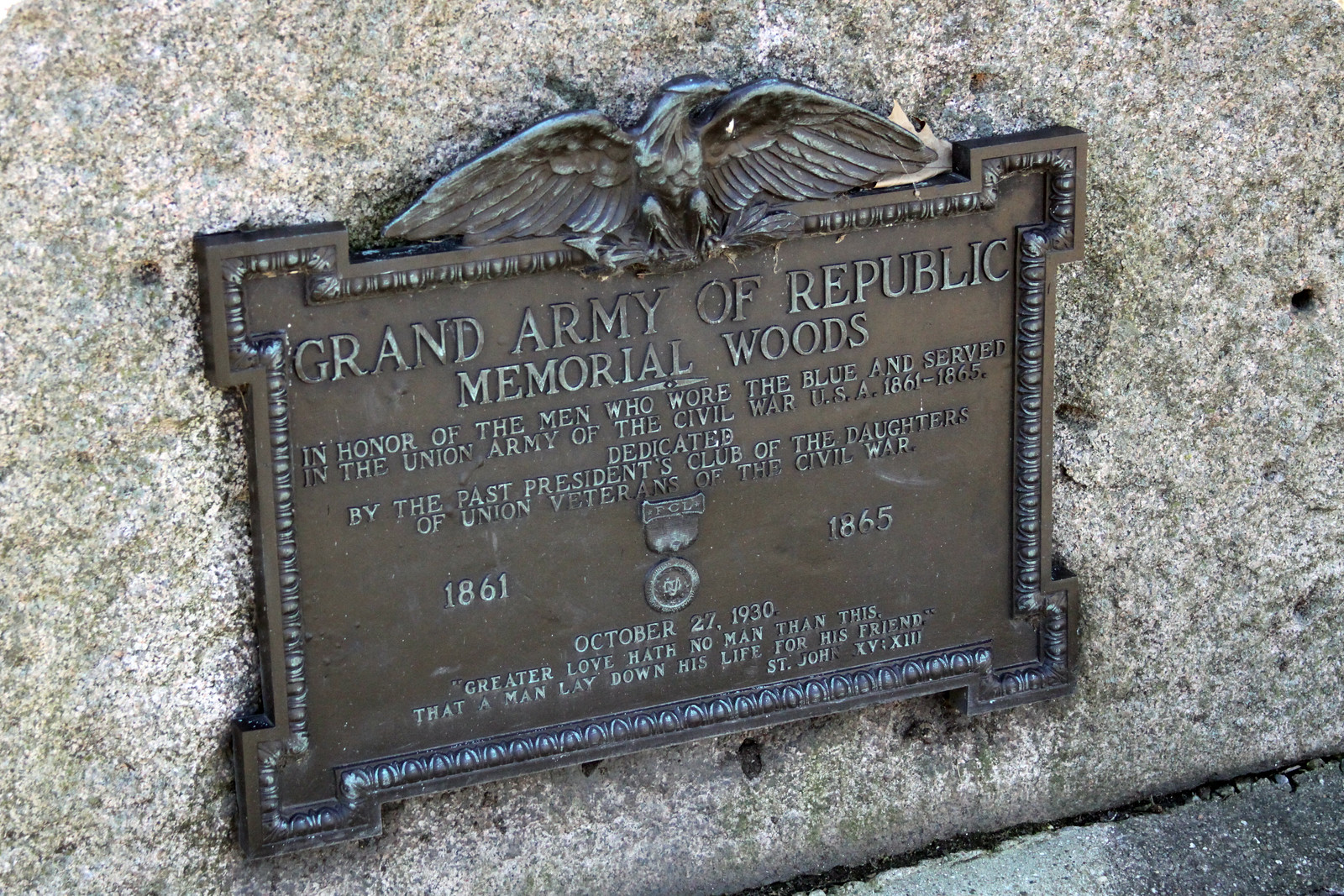The image features a commemorative bronze plaque mounted on a rugged limestone or concrete wall. The plaque is square with elegantly extended corners, and at the very top, there's a striking black metal eagle with its wings spread wide. Centrally inscribed in silver letters, it reads "Grand Army of the Republic Memorial Woods." Beneath this, the inscription honors "the men who wore the blue and served in the Union Army of the Civil War." The plaque also features a central image of a medal, flanked by the years "1861" on the left and "1865" on the right, marking the duration of the Civil War. Below, the text indicates that the dedication was made by the Past Presidents Club of the Daughters of Union Veterans of the Civil War, with the dedication date of October 27, 1930. The plaque concludes with a poignant quote: "Greater love has no man than this, that a man lay down his life for his friend."